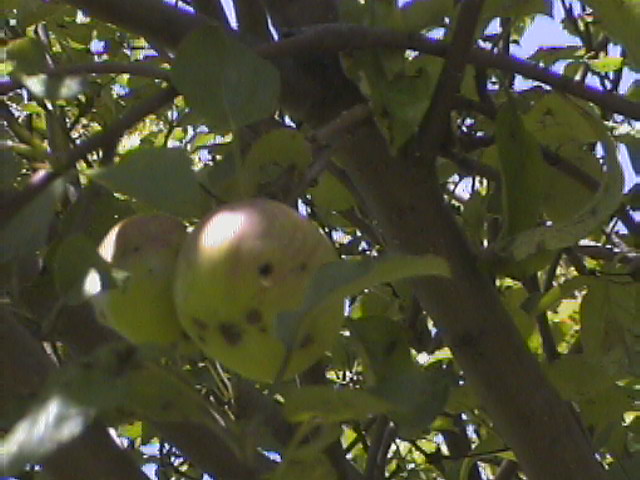This is a horizontal, close-up photograph of an apple tree taken from below, looking up into a dense canopy of light green leaves and grayish-brown branches. The image is slightly blurry and pixelated, giving it a grainy appearance. Dominating the left side of the frame are two unripe apples, predominantly light green with red streaks, and showing signs of pest damage and dark spots, possibly indicative of fungal infections or wormholes. One of these apples has a sunken spot. Despite the general dimness of the scene due to the foliage blocking out much of the sunlight, both apples exhibit bright reflections as if they're catching light. In the background, through the thick foliage and branches, glimpses of a blue sky can be seen, adding a subtle contrast to the green and brown tones dominating the image.